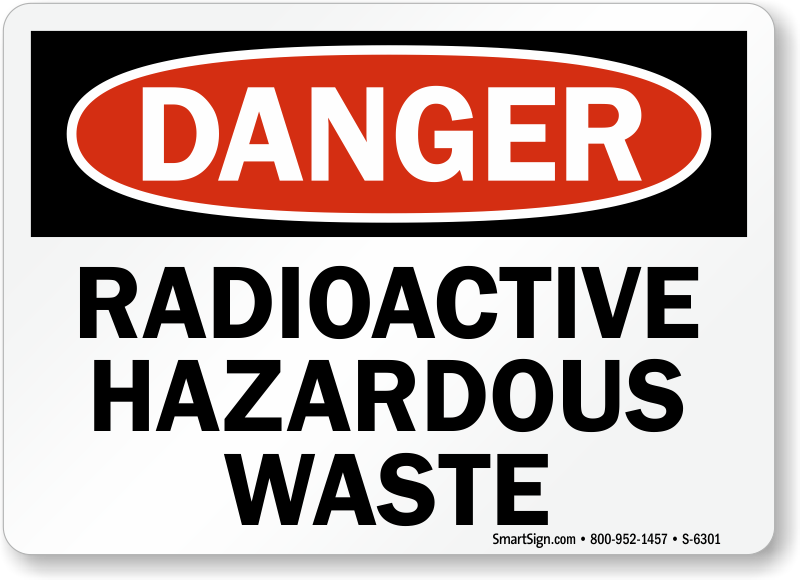The image showcases a rectangular, eye-catching warning sign with a white background. Prominently positioned at the top one-third of the sign is a black banner. Within this banner, a bold red oval with a white border contains the word "Danger" written in large, white, capital letters. Below the black banner, on the white background of the sign, the message "Radioactive Hazardous Waste" is clearly displayed in black letters. At the bottom-right corner, the sign includes the manufacturer's information: "smartsign.com," a contact number "800-952-1457," and the model number "S6301." This detailed and distinctive design ensures the sign is highly visible and easily readable, effectively warning of the serious hazards associated with radioactive waste.